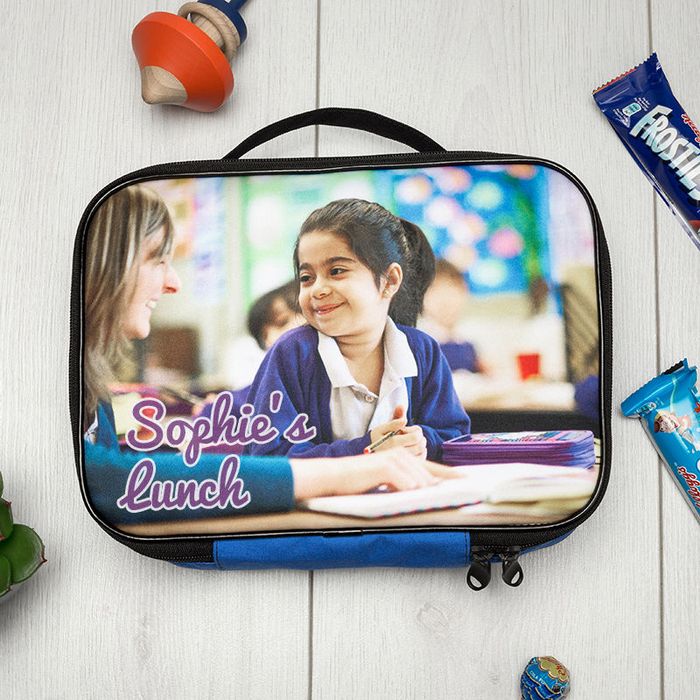In this detailed image, a lunchbox is prominently positioned at the center of a light gray wooden table with subtle white and gray detailing that mimics wood paneling. The lunchbox itself has bright blue edges, a black zipper, and a black handle. On the front of the lunchbox, there's a printed photograph featuring a little girl with her black hair in a ponytail, wearing a white shirt and a light purple jacket, who is smiling at a woman with thin blonde hair, likely a teacher, who appears to be explaining something. The phrase "Sophie's Lunch" is written in purple cursive letters above the picture. Surrounding the lunchbox, there are various snacks: a dark blue package with white lettering that says "Frosties" or "Frosted" and a light blue package featuring a Keebler elf and "Kellogg" in red. Other items scattered around include a Rice Krispie treat, a toy, and part of a plant. The background details and the positioning of the items suggest a casual, everyday setting.